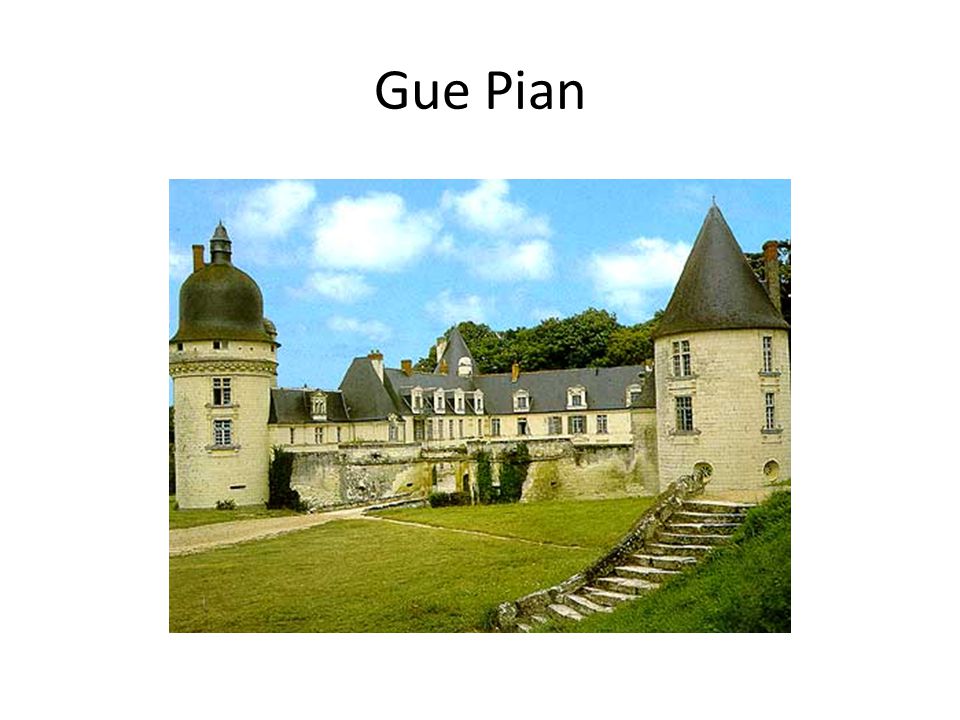The image depicts a historic French chateau with the text "Guy-Pian" prominently displayed above its entrance. The main structure features white bricks and is characterized by two distinctive towers, one on either end. The right tower has a pointed cone roof with an old stone staircase leading up to it, while the left tower boasts a rounded, bell-shaped roof with a point at the top, and a chimney on its side. Both towers feature ornamental trim and windows, enhancing their architectural elegance. A long connecting building sits between these two cylindrical towers, with the rooftops of all parts of the chateau being gray in color. In the foreground, a lush green lawn is delineated by a path and a road leading over a bridge to the entrance of the chateau. The lawn also includes some dark greenery along a wall. In the background, the tops of trees can be seen peeking above the roof, under a blue sky filled with white clouds.